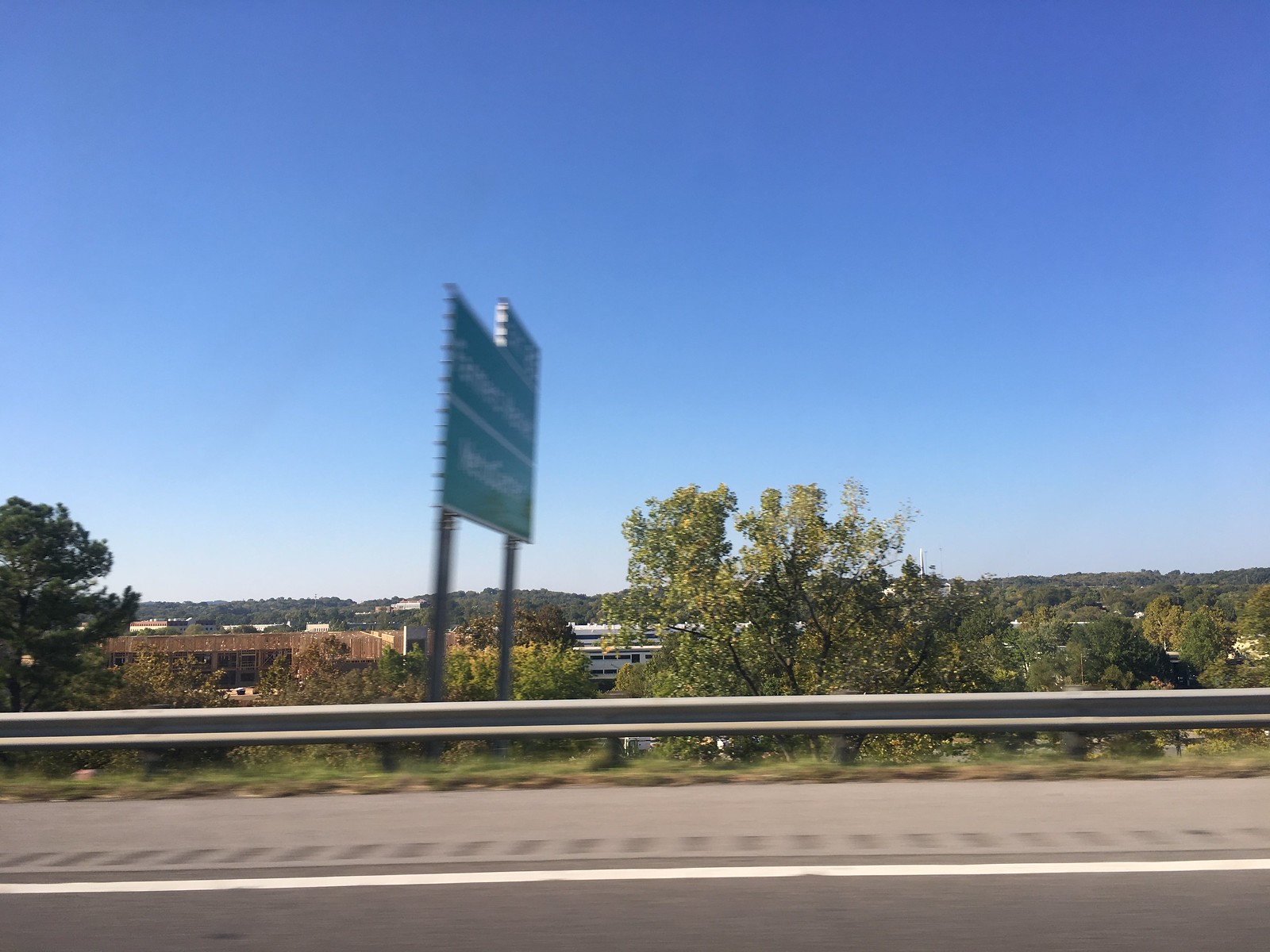In this swiftly captured image, we see a scene taken from a moving vehicle, as if the photographer had glanced out the side window and snapped the shot in a fleeting moment. The background is sharply in focus, revealing a row of tall shrubs and small trees, with one prominent tree standing out clearly. Below, a gray railway runs parallel to the road, hinting at the presence of a nearby train route. Although the road itself is only partially visible, the distinct strips designed to alert drivers of drift are noticeable. In the distance, there is a green sign with white text, likely indicating an upcoming exit or direction, though it appears slightly blurry due to the quick nature of the photograph. The overall scene captures the brief, transitory essence of a journey along this roadway.